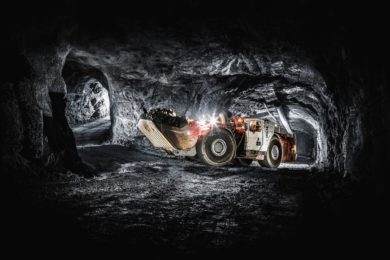This photograph captures an interior scene of a narrow, dimly-lit coal mine tunnel illuminated by the bright headlights of a gray-brown front loader with black tires. The loader, heavily laden with a full scoop of coal that piles above its bucket, is positioned at a junction between two passageways. The vehicle, emitting light, seems to be making a right-hand turn upwards into a new tunnel, with its path leading from a darker area towards a lighter section of the cave. Above, pipes run along the ceiling, contributing to the mine's industrial setting. Further back, a warmer light casts partial illumination. The rustic, constrained atmosphere of the mine is punctuated by the stark contrast of the loader’s headlights against the shadows.